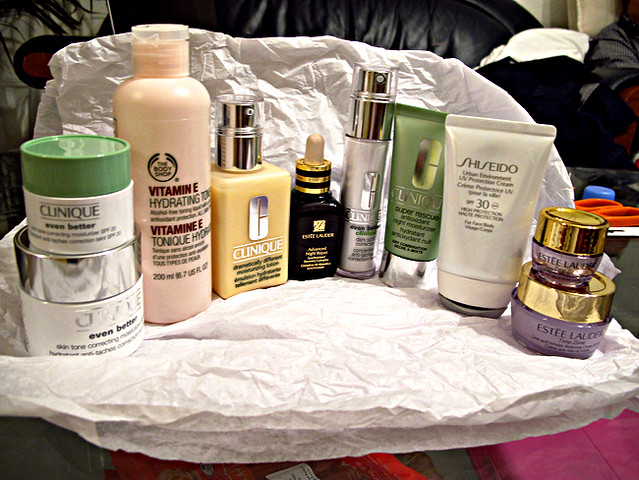The photograph showcases a meticulously arranged display of various beauty products atop a table adorned with crinkled, white tissue paper. On the far left, there are several jars of Clinique face lotion, easily recognizable by their distinct packaging. Adjacent to them is a pink bottle of The Body Shop's Vitamin E Hydrating Toner, characterized by the Body Shop logo and the Vitamin E label in red font.

Next in line is a square, yellow bottle of Clinique's iconic Dramatically Different Moisturizing Lotion, featuring its famous silver "C" emblem. To the right of this is an Estee Lauder product, identifiable as an Advanced Night Repair serum, housed in a typical eye dropper bottle.

Continuing to the right, more Clinique items are visible alongside a white bottle of Shiseido's sunscreen. The display is completed by two Estée Lauder night creams in their signature purple and gold jars. The overall presentation of these diverse beauty products creates a visually appealing and organized showcase.